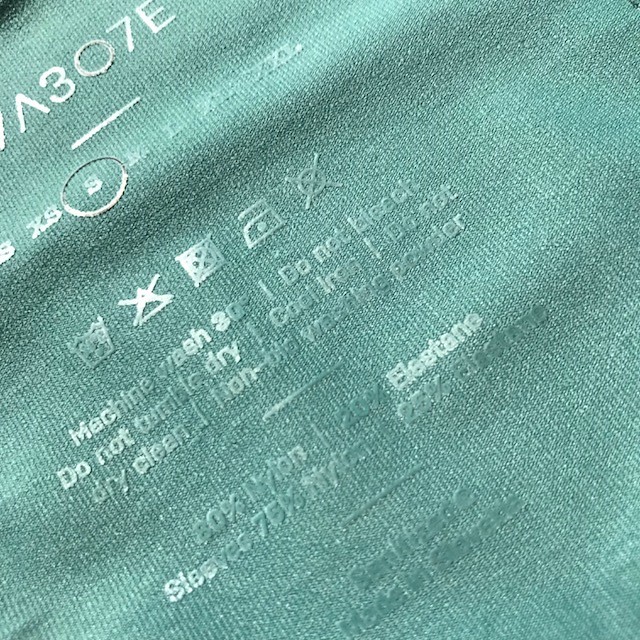A high-resolution, close-up shot of a fabric's care label dominates the frame, angled slightly to the right. The material appears greenish with a somewhat faded hue, indicative of multiple washes. At the very top of the label, an inverted V-shaped "30" is visible—potentially part of the brand's name or logo. Directly below, a circled "S" highlights the size as small, flanked by XS, M, and L indicating other available sizes in a subtle, washed-out print. 

The care instructions are prominently displayed, albeit slightly faded, detailing the recommended maintenance procedures: machine wash, avoid bleaching, do not tumble dry, use a cool iron, and dry clean if necessary. Prohibited actions are marked with clear Xs. Further down, the label lists the fabric composition, mentioning nylon and elastane, with a note that the sleeves consist of a different material, though specific details are obscured by wear and tear. The overall appearance suggests a well-loved garment, providing insight into both its quality and longevity.